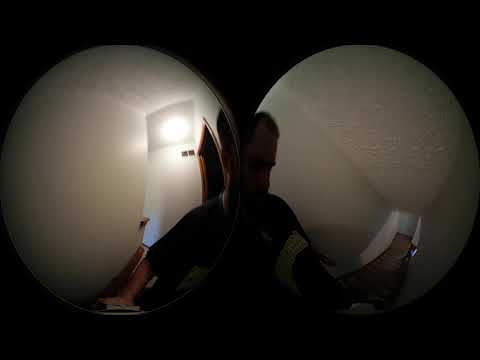The image features a horizontally aligned, almost-square format with a solid black background. At the center, two circular shapes—resembling overlapping peepholes or binoculars—reveal a slightly blurred scene set in a dimly-lit indoor area, likely a hallway or room. 

In these circles, a textured wall in shades of white, beige, or gray forms the backdrop. The left circle showcases part of the man's right arm and sleeve of his short-sleeved, black shirt, which has indistinct green markings. This circle also hints at a hallway leading towards a light source. The right circle captures the man's face looking slightly downward to the right, emphasizing his short brown hair, a potential shadow-covered facial hair, and his left arm holding a blurred object. Below the circles, we see what appears to be brown-colored stairs descending, contributing to the overall indoor aesthetic.

Positioned centrally in both circles, the man’s right arm rests on a piece of paper placed on a table or desk, adding to the impression that the setting might be a residential space, possibly at the top of a staircase. The absence of text within the image accentuates a unique perspective, potentially achieved through stitching together two images taken through a peephole, yielding a convex, vignette-like effect.